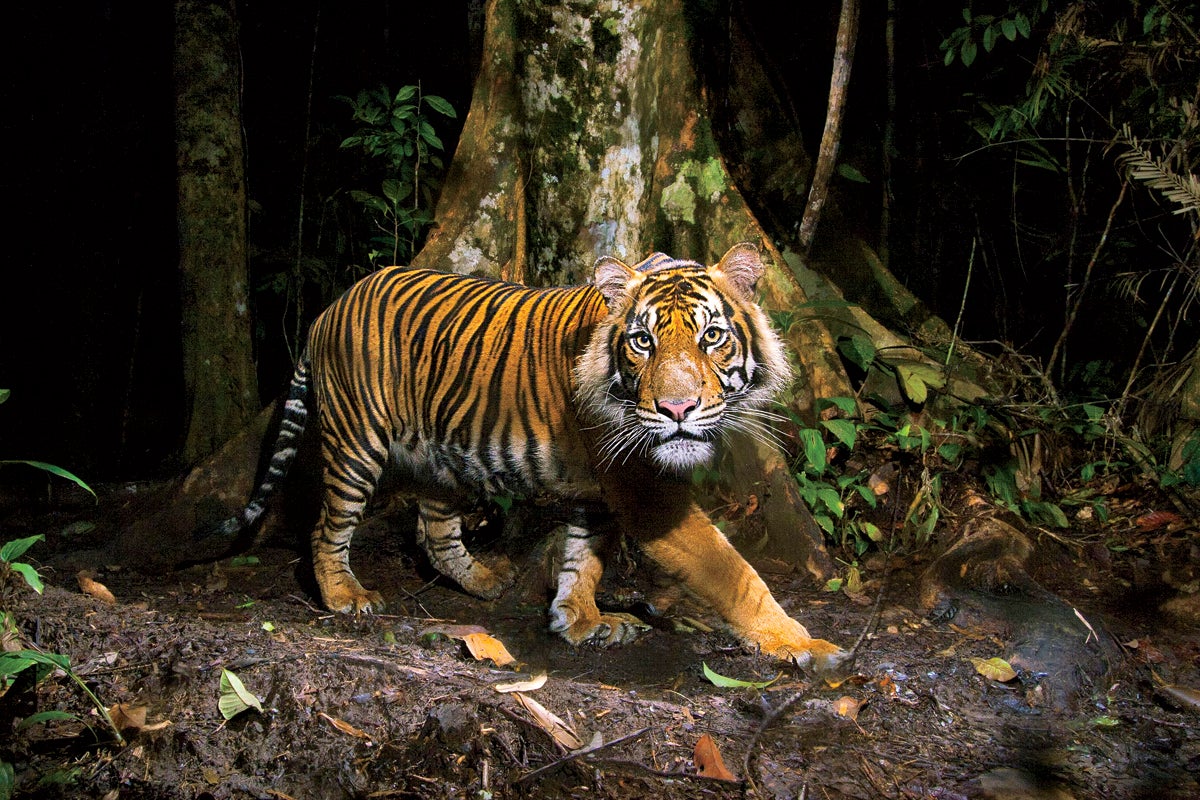This image features a striking Bengal tiger prominently positioned in the center, walking from left to right along a damp, muddy dirt path in a dense forest. The tiger's gaze is fixed directly on the camera, capturing its intense, yellow eyes. Its powerful, stocky body displays a typical orange and black striped pattern, with a white and black striped underbelly and tail. The face, framed by rounded ears, combines orange fur and black striping with white accents around the eyes, chin, and a light brown nose. The scene is set at the base of a large, old tree with an extensive root flare, possibly displaying white mold or fungus. Additional trees compose the background, adding depth and emphasizing the natural habitat. The tiger does not appear aggressive but rather curious, as it continues its walk with its front right paw extended forward. The overall atmosphere conveys the raw beauty and majesty of the Bengal tiger in its natural environment.